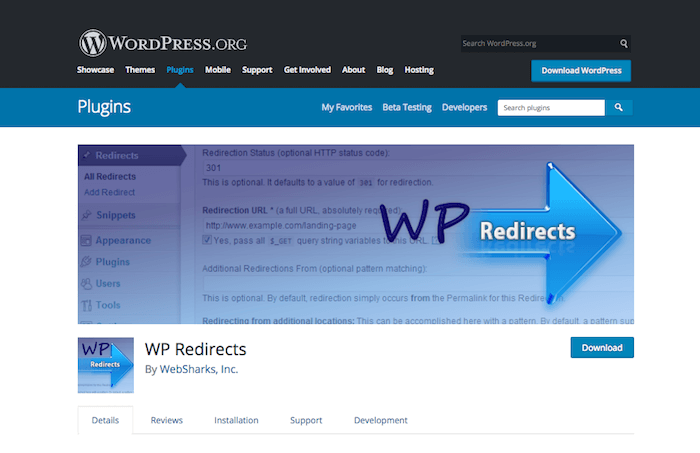This is a detailed screenshot of the WordPress.org website. At the top of the screen, there is a navigation bar set against a black background, featuring the WordPress logo—a white "W" inside a black circle. The navigation options include: Showcase, Themes, Plugins, Mobile Support, Get Involved, About, Blog, and Hosting. Below the navigation bar is an aqua-colored button labeled "Download WordPress."

Further down the page, there's an aqua-colored section titled "Plugins." This section includes subcategories such as My Favorites, Beta Testing, Developers, and Search Plugins. Beneath this, there's a faintly visible box with text about redirection status. The text explains that the default value of redirection is optional and currently set to "WP."

Prominently featured is a large blue arrow pointing to the word "Redirects." Below this, there's a smaller box labeled "WP Redirects" accompanied by an arrow icon. Next to it, text reads "WP Redirects by websharks.inc."